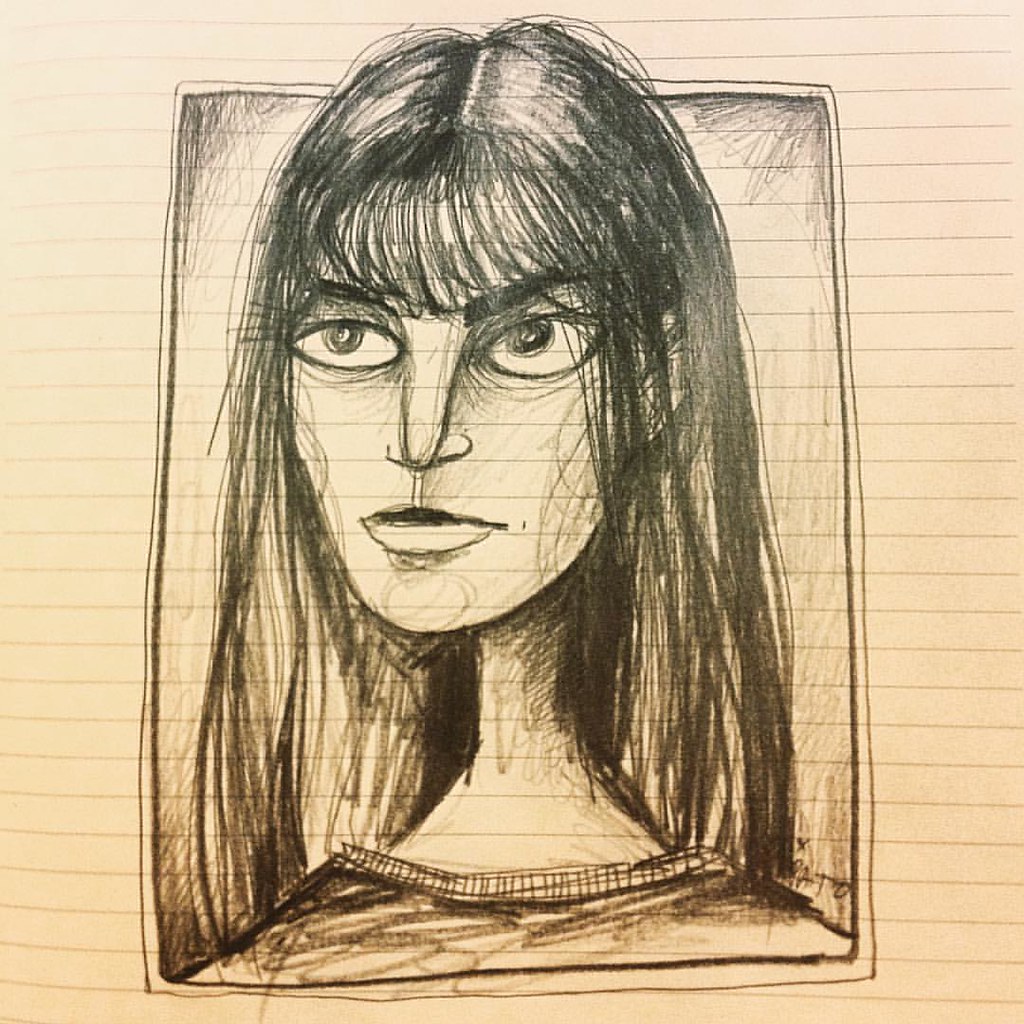The detailed pencil sketch, set against a backdrop of pale-colored, rolled paper resembling a page from an exercise book, features a woman with strikingly elongated facial features. Her straight, center-parted hair cascades down her back, framing her face. Large, expressive eyes, reaching the sides of her face, are accentuated by long lashes and straight eyebrows visible beneath her bangs. Her angular nose adds to the distinctive character of her face. Despite the simple medium, the artist has meticulously crafted each detail, resulting in a captivating portrait that draws the viewer's gaze straight into hers.